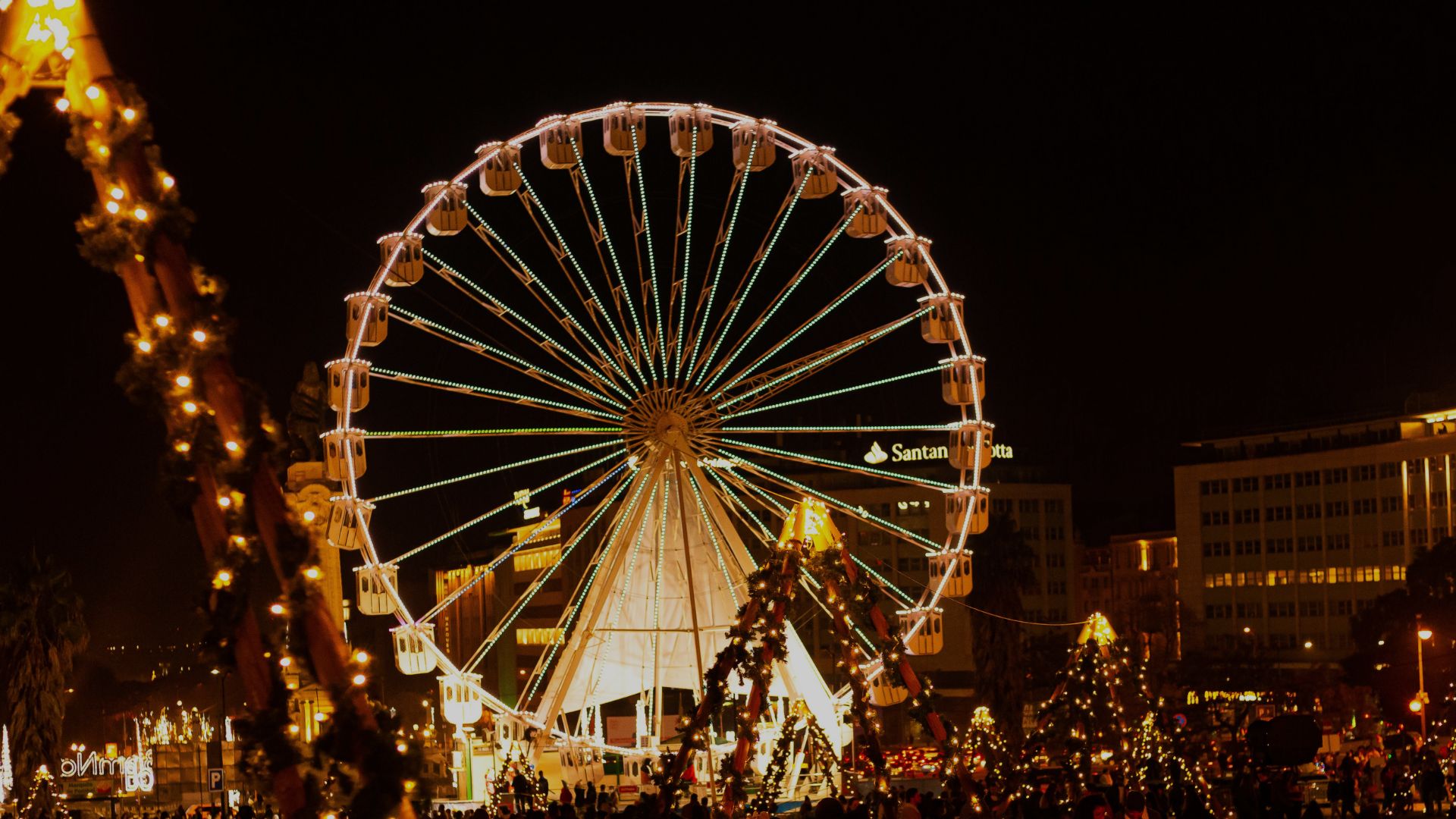The image captures a vibrant nighttime scene centered around a large Ferris wheel adorned with horizontally running green lights and individual ride seats at their ends. The Ferris wheel stands prominently, roughly half the height of the surrounding 10-story buildings, including one with a visible "San Tan" sign. The sky is a pitch black, emphasizing the illuminated elements. In the foreground and background, wood slanted pyramid structures resembling Christmas trees are festively decorated with garlands, yellow Christmas lights, and evergreen branches or pine needles, creating a warm holiday atmosphere. The left side of the image features glowing light strings running from top to bottom, while the right side showcases additional lit-up buildings and cityscape elements, further enhancing the celebratory mood of this town square fair.